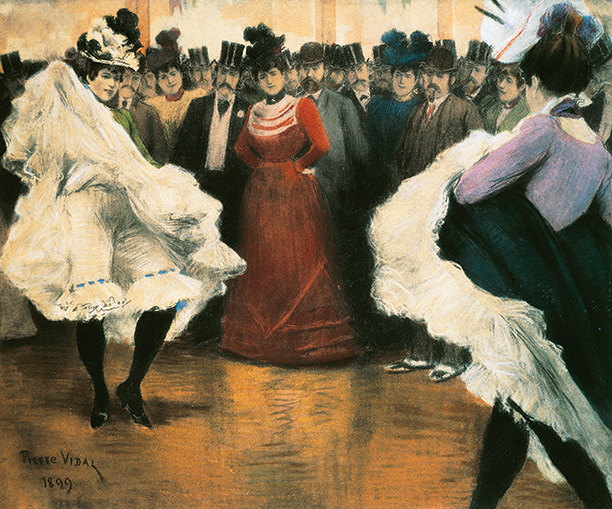This vibrant painting by Pierre Vidal, dated 1899, captures an energetic scene at an elegant dance hall, rendered with an impressionist touch. Central to the composition are two can-can dancers, positioned in the foreground, facing each other and performing with spirited confidence. The dancer on the left, visible from the front, confidently lifts her long dress to reveal black stockings and petticoats beneath. She wears a hat adorned with white and black feathers. Opposite her, the dancer on the right, viewed from behind, mirrors this action, lifting her dress to reveal similar attire.

The scene is set on an orange and black checkered floor, amidst a crowd of spectators dressed in formal 19th-century attire. The men predominantly wear bowler hats, top hats, and tuxedos, while the women are clad in long, elegant dresses and elaborate feathered hats. Notably, a woman in a long red dress with a black feathered hairpiece stands out in the center of the crowd. The background is awash with light brown and orange hues, enhancing the vibrancy of the dynamic dance competition. The artist's signature, "Pierre Vidal, 1899," is inscribed in black text at the lower left corner of the painting.